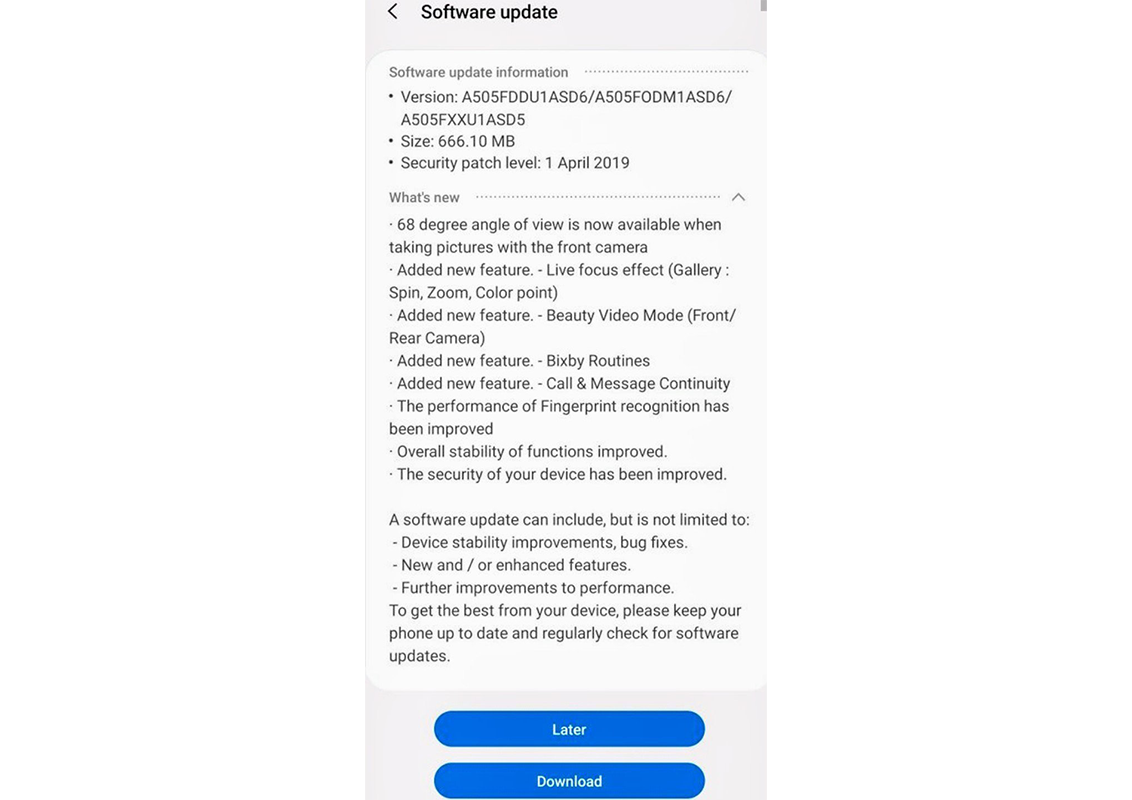The screenshot captures a software update notification on a cell phone. At the top left, it displays "Software Update" accompanied by a back arrow, indicating the option to return to a previous screen. Below this header is a divider section titled "Software Update Information."

The lower part of the screenshot includes two blue buttons: one labeled "Later" and the one beneath it reading "Download." The main information section informs about the update, mentioning that it includes 35 security patches.

What's new in the update features prominently:
- **Enhanced Viewing Angle:** A 60-degree angle of view adjustment.
- **Live Focus:** Introduction of the live focus feature for improved photo quality.
- **2D Video Mode:** Addition of a new 2D video mode.
- **Secure Picture Routine:** Integration of a new secure picture routine.
- **Call and Message Continuity:** Feature added for continuous call and message functionality.
- **Improved Fingerprint Recognition:** Enhanced performance for fingerprint recognition.
- **General Enhancements:** Improved overall stability of functions and device security.

This update appears to be associated with an Android version, as indicated towards the end of the screen. Additionally, it notes that the software update may include device uploading or enhanced features.